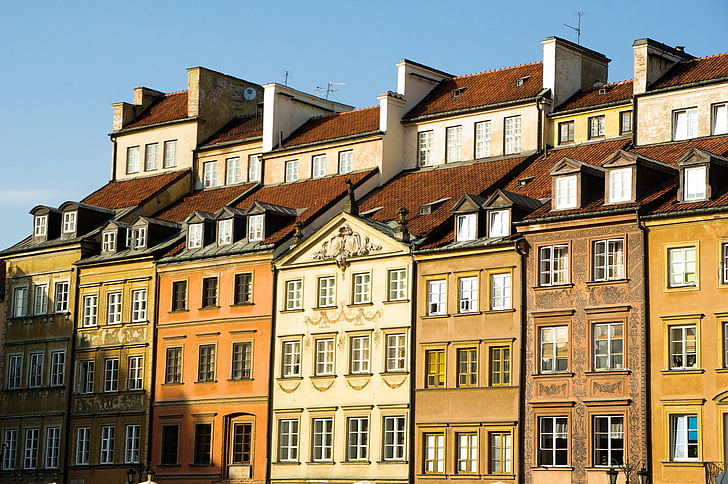The photograph captures a striking row of six multi-story houses set against a cloudless blue sky, exuding a distinct European, possibly Eastern or Northern, architectural charm. From left to right, the facades display a palette ranging from dark yellow to orange, cream, tan, brown, and light orange. Each of these houses features three visible stories with a fourth penthouse-like level that sits atop their slanted brown tiled roofs. The first two houses, in dark yellow, have uniform white window frames, while the orange house next to them has dark brown frames. The central cream-colored building is adorned with intricate eaves and white window frames, providing a decorative highlight. Adjacent to it, the tan house stands out with its yellow window frames, while the subsequent brown house displays consistent white window frames. The final house, a light orange, maintains the uniformity with white-framed windows. Each building's roof might include gabled windows, skylights, or antennas, hinting at a well-populated urban area. The sunny day accentuates the vividness of the colors and the architectural details, suggesting a vibrant neighborhood preserved in its historic, old-world grandeur.